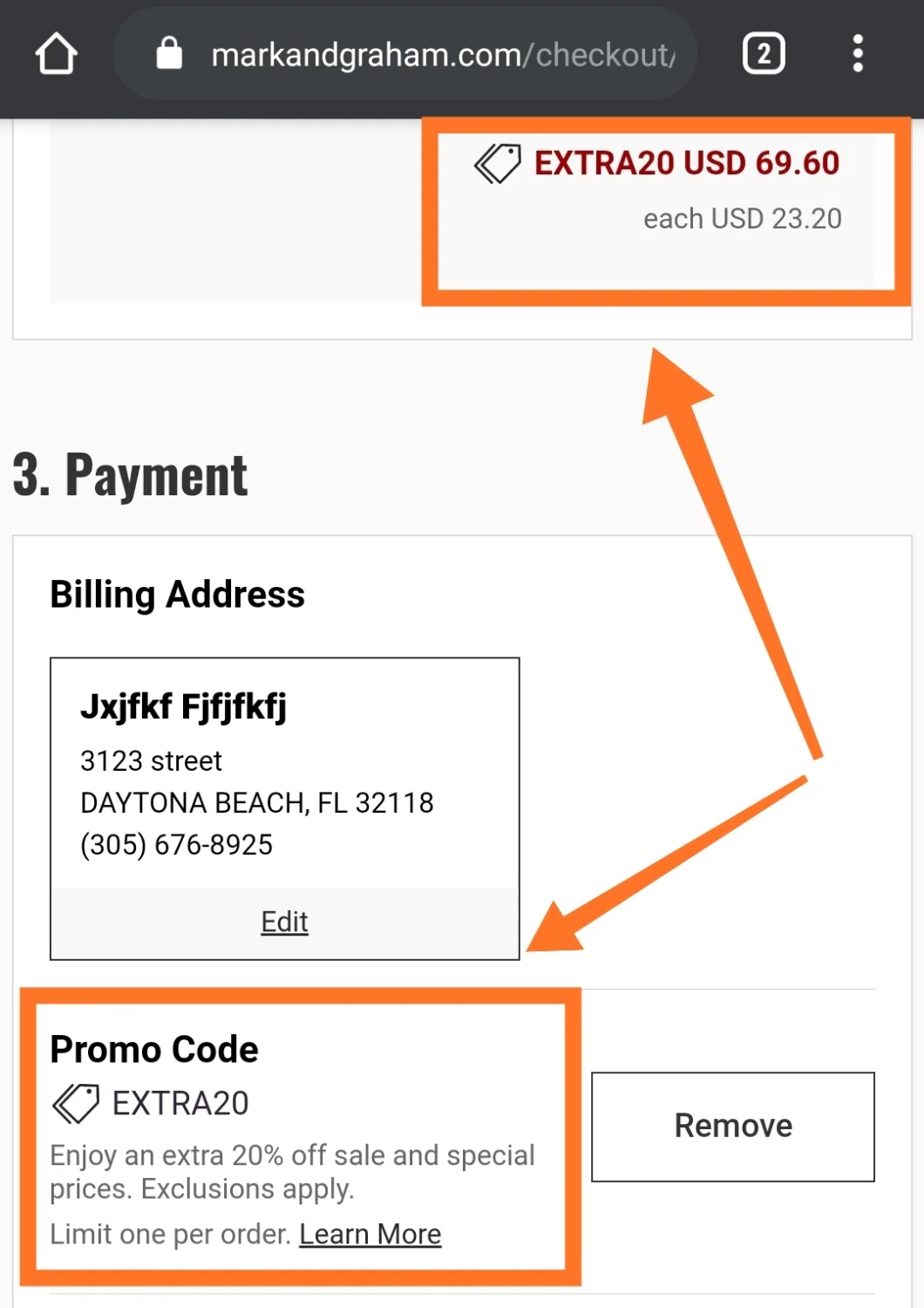The screenshot displays a user navigating a mobile version of the website markandgram.com, specifically on the checkout screen. The site appears to be under construction, as indicated by the presence of placeholder text. The visible portion of the checkout process highlights step three and partially reveals step two. In step two, a summary suggests that three items have been purchased, totaling an extra $69.60 USD, with each item priced at $23.20 USD.

The payment section below includes dummy text filled into the billing address fields. Additionally, there is a promo code area containing the text "extra 20," which relates to a promotional offer of 20% off a sale with special prices, noting that exclusions apply and there is a limit of one code per order. The promo code section is further emphasized with orange boxes and arrows drawn around the relevant text.

The top navigation bar of the browser is dark, indicating the use of Google Chrome, and a home button is visible on the left side. There is at least one other tab open, but its content is not disclosed. The main page has a white background with predominantly black text, creating a straightforward and clean visual presentation.